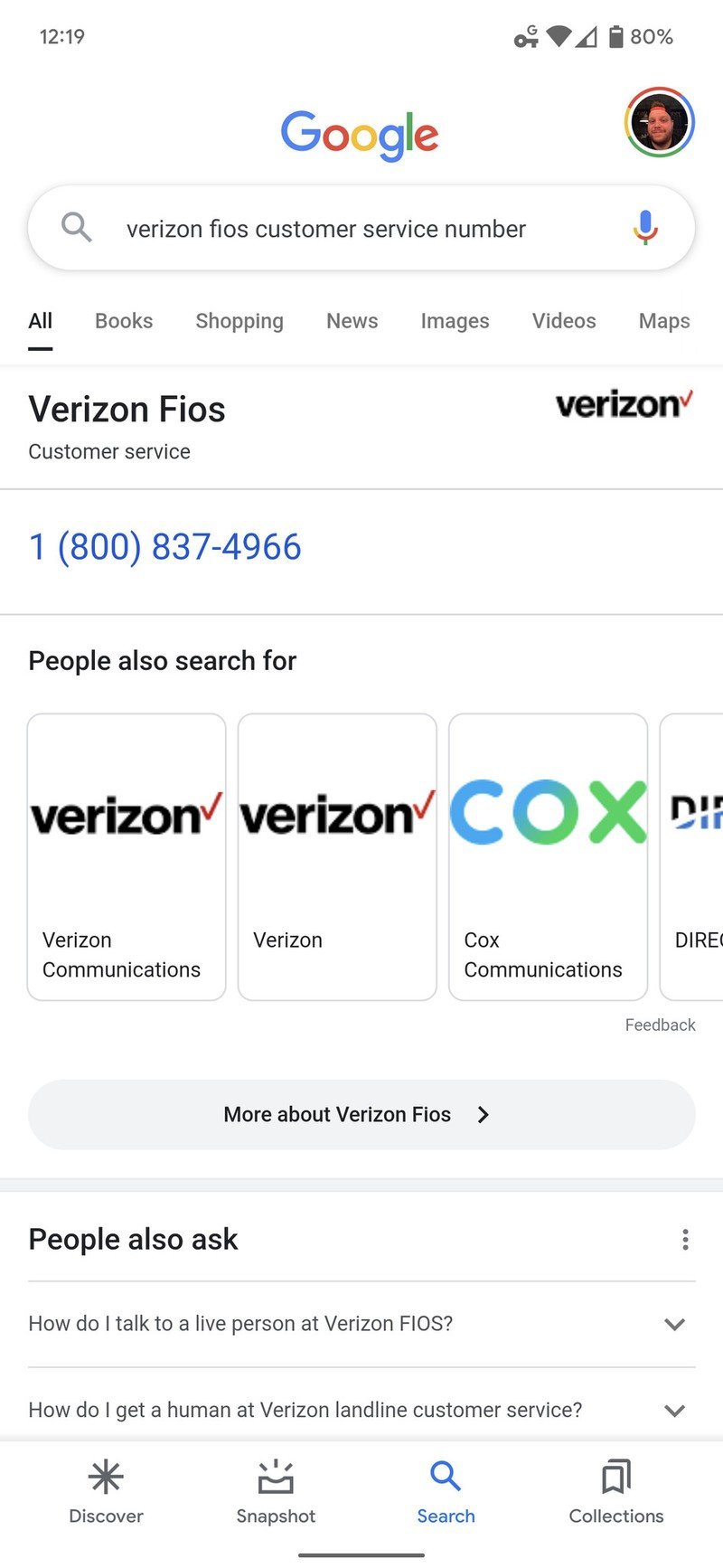This screenshot, captured from a smartphone, vividly details various on-screen elements. In the upper-left corner, the time prominently reads 12:19. Opposite this, in the upper-right corner, the icons indicate an active Wi-Fi connection and a battery at 80%. Central to the image, a circular profile picture displays a young man with a beard, dark hair, and fair complexion. This profile photo is embedded within the Google interface. Below, the iconic Google logo is presented in large, clear text, with a search bar directly underneath.

Within the search bar, the phrase "Verizon Fios customer service number" can be seen. Under this, a navigational bar features various options—All, Books, Shopping, News, Images, Videos, Maps—indicated in bold black text. Dominating the screen, a search result for "Verizon Fios customer service" displays the number 1-800-837-4966 in bold text. Supporting this, the suggestion "People also search for" is listed in blue text directly below. The screenshot effectively captures a snapshot of a detailed search query within the Google app on a smartphone.